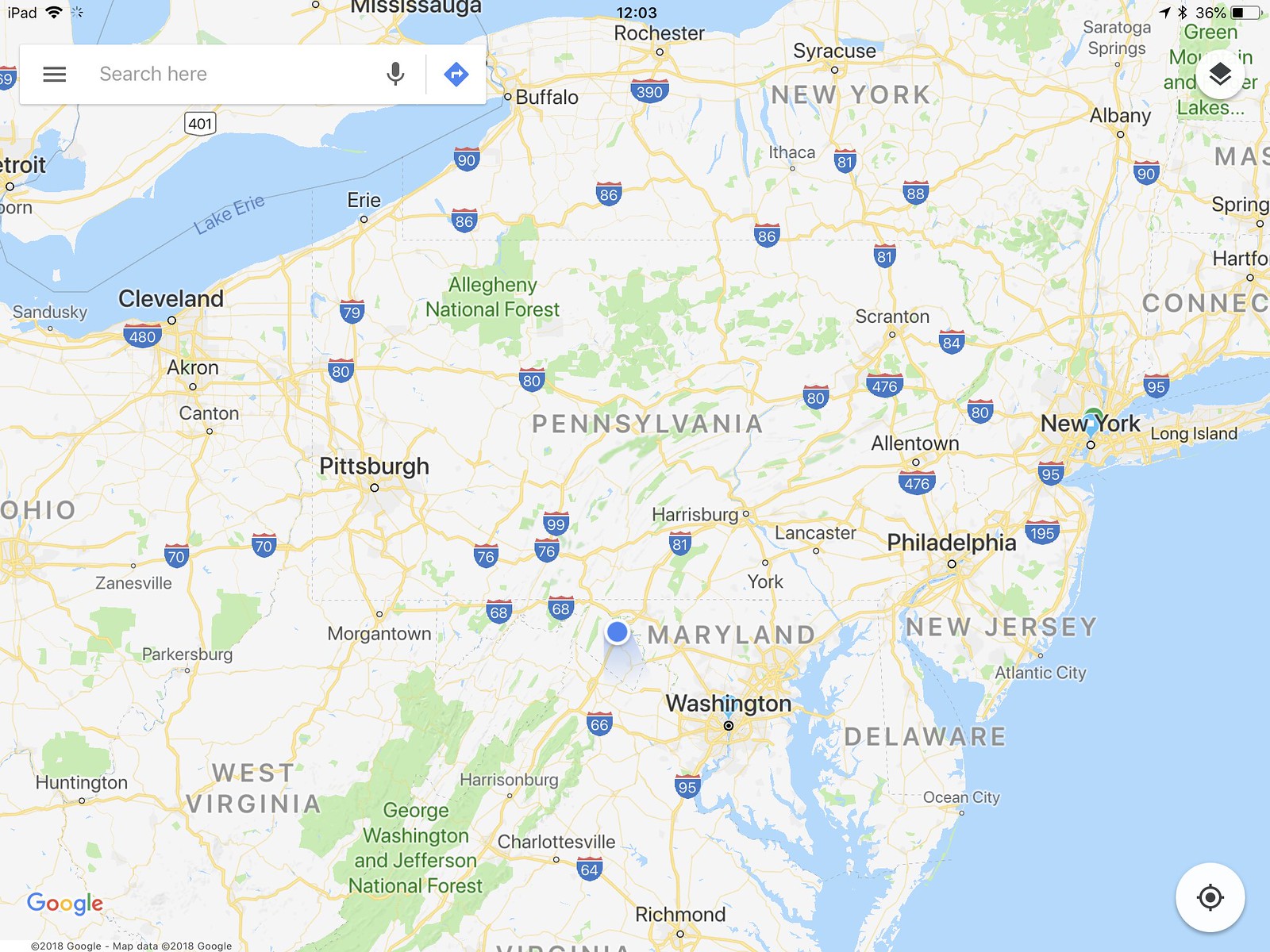This image is a detailed screenshot of Google Maps viewed on an iPad, depicting the northeast region of the United States. From a top-down perspective, the map prominently features several states including Connecticut, New York, Pennsylvania, West Virginia, Ohio, Delaware, Maryland, and New Jersey. The map is visually coded with various colors: bodies of water like the Atlantic Ocean and Great Lakes (including Lake Erie) are rendered in blue, forests and national parks are shown in green, and city areas are marked in white. Yellow lines represent major interstate highways, which are clearly labeled with blue interstate signs for easy navigation.

The map also includes detailed city markers, extending up to Rochester and Syracuse in New York, and as far south as Richmond, Virginia. Additionally, tech details such as the iPad's 36% battery indication, active Bluetooth and location settings, and a strong Wi-Fi connection, are visible. The screenshot captures a timestamp of 12:03, and the interface includes a search bar in white, located at the top, enabling quick searches and navigation. This comprehensive map provides a clear and informative layout of the region, ideal for planning travels or identifying specific geographic details.